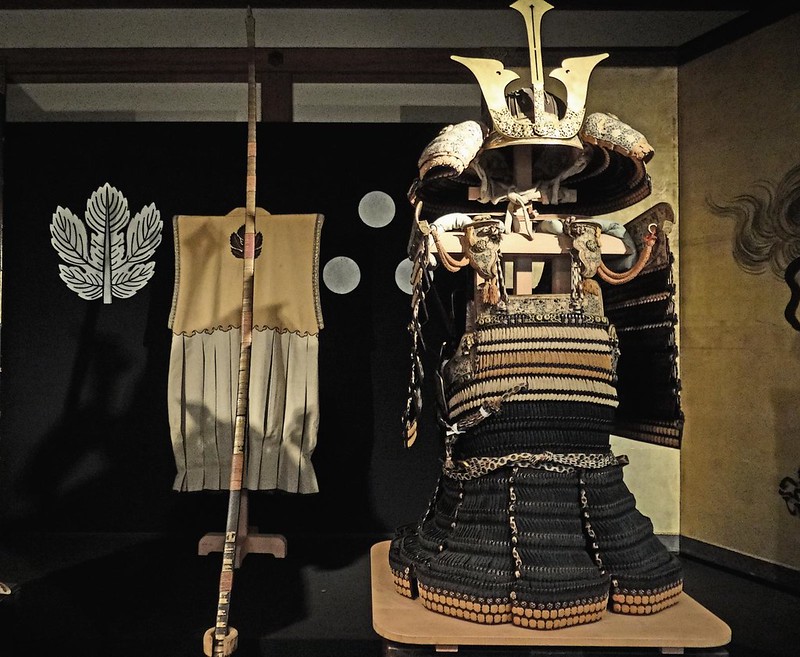This photograph captures an exhibit likely located in a history museum, showcasing a full set of traditional samurai armor positioned prominently on the right. The armor includes a distinguished helmet with three metal prongs extending from the center, adorned in gold with orange ropes. The body armor features intricate beadwork with hues of black at the bottom and faded orange and beige stripes above. The ensemble is mounted on a wooden base. To the left of the armor, a katana, encased in a wooden or bamboo sheath, stands supported by a wooden pole, with a rectangular beige flag hanging behind it, possibly representing the samurai. The backdrop is predominantly black, decorated with a white leaf design on the left and a pattern of three white dots arranged in a triangle to the right. Additionally, a gold and brown Japanese room divider is partially visible to the far right, complementing the Japanese theme of the exhibit.